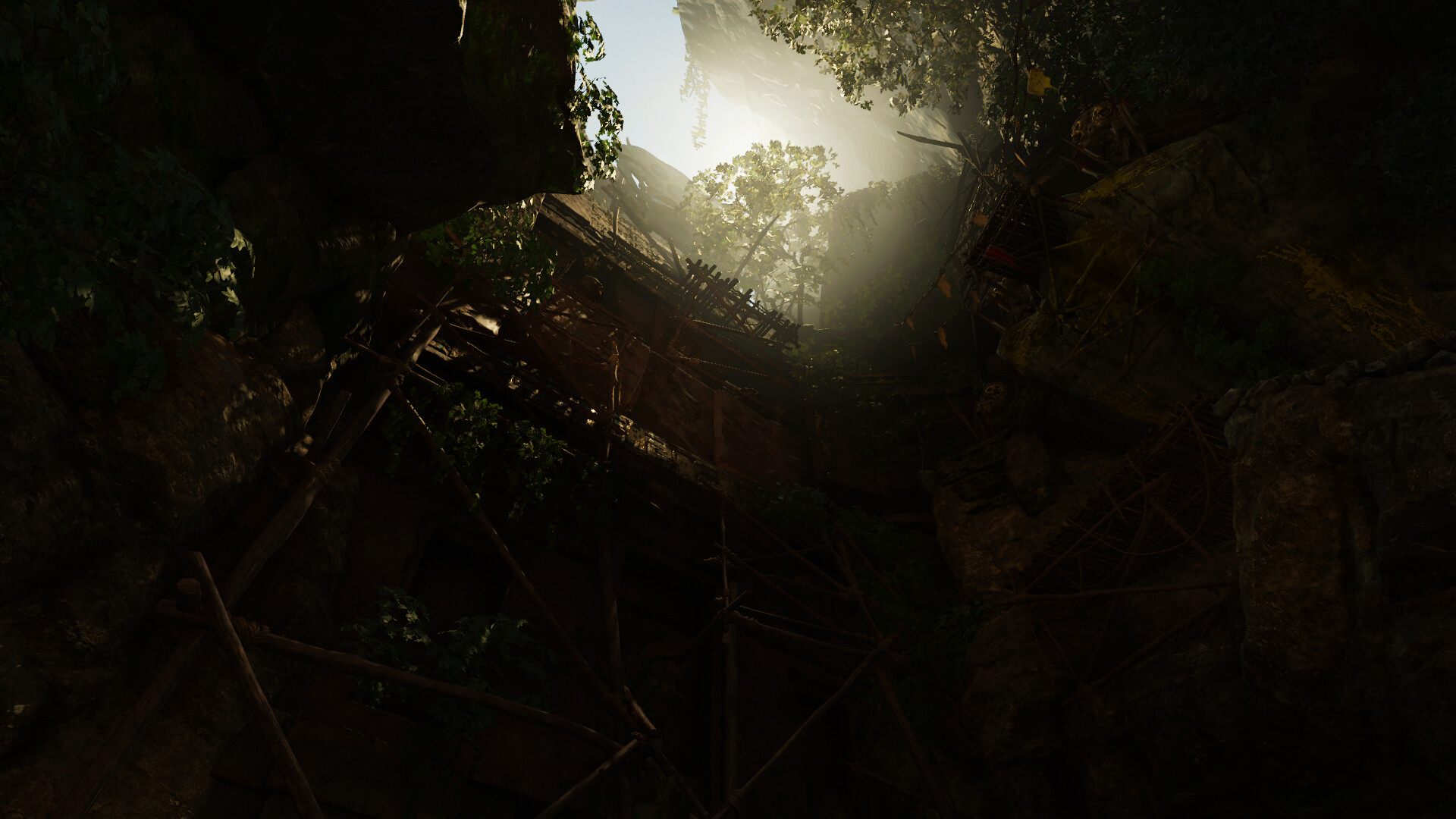The image appears to be taken from ground level, looking upwards from within a darkened, cave-like environment. Surrounded by large boulders or possibly the foundation of an ancient structure, the scene is bathed in muted, dark shades of brown and green. There is a wooden structure or primitive ladder on the side, composed of large sticks, providing a pathway towards the light. Above, a small portion of the sky gleams a beautiful blue, framed by green leaves and tree branches that partially obscure the view. Sunlight streams down through this opening, illuminating the upper center of the image. The hints of a mountainside or cliff edge add to the rustic forest scenery. The overall impression is one of looking up from the subterranean depths of a forest landscape, drawn towards the bright slice of sky and sunlight overhead.